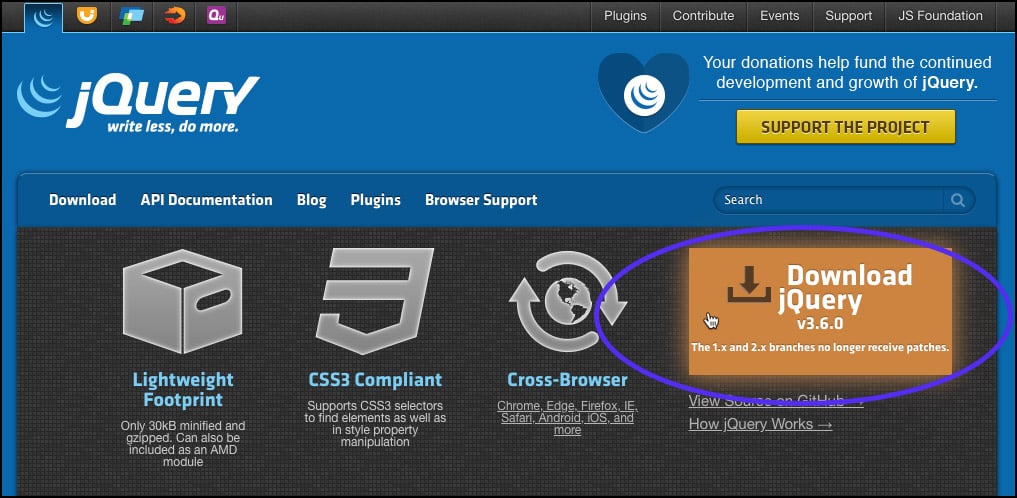In this image, the central theme is a blue background adorned with various elements and informative boxes. 

1. **Top Section:**
   - The image features a black box positioned at the top, near the left corner, creating a little rise in the blue area, forming a box with rounded lines.
   - Inside this black box, there's a yellow semicircle containing a 'J' symbol, and next to it, a blue box with green content.
   - Adjacent to these, there's an orange circle with a right-facing black arrow, followed by a purple square lying horizontally, resembling a 'P'.
   - Text labels such as "Plugins", "Contribute", "Events", "Support", and "JS Foundation" are displayed.

2. **Main Body:**
   - The primary section of the image is dominated by a big blue section with three curved lines, captioned with "jQuery: Write Less, Do More."
   - Centrally, a large blue heart symbol is present, encompassed by a white circle with curved blue lines.
   - Below this, a text reads "Your donations help fund the continued development and growth of jQuery."

3. **Call-to-Action:**
   - Beneath the main section, a bright yellow button is marked "Support the Project."

4. **Additional Information:**
   - Another blue box follows, listing "Download", "API Documentation", "Blog", "Plugins", and "Browser Support".
   - There's also a substantial search box for navigational purposes.

5. **Feature Highlights:**
   - A large black box showcases key features like "Lightweight Footprint: only 30 KB used," "CSS3 Compliant," and "Cross-Browser Compatibility" with logos for Chrome, Edge, Firefox, Safari, and Android.

6. **Version Information:**
   - At the bottom, a brown box encircled by a blue ring emphasizes "Download jQuery Version 3.6.0," with an open square and a down arrow icon.
   - It includes a notice of a white hand icon stating that the "1.x and 2.x branches no longer receive patches," followed by two questions with underlines beneath them.

This image aims to visually communicate detailed information about jQuery's features, support, and updates.